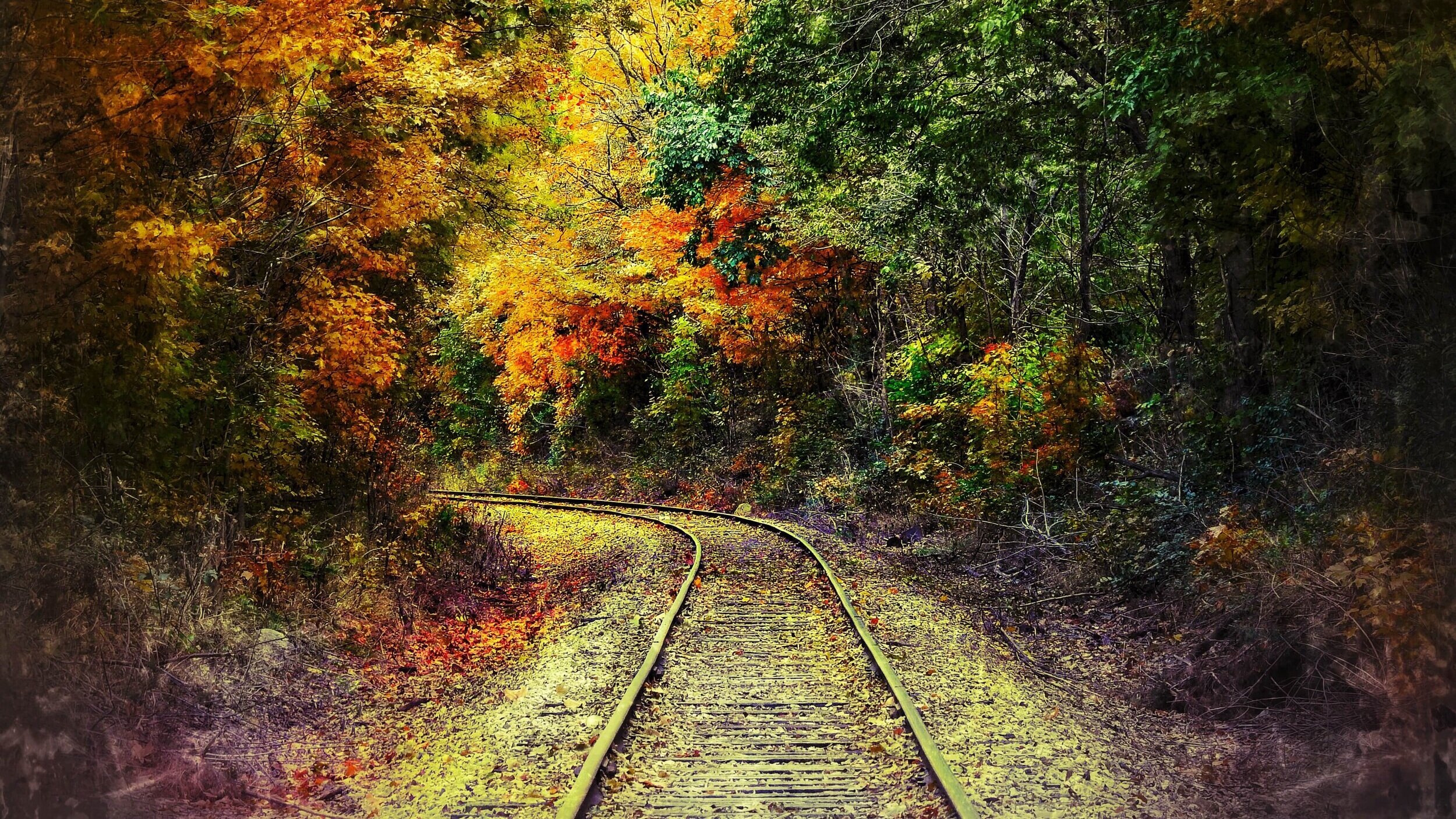The image depicts a tranquil autumn landscape centered around a railway track that stretches forward from the foreground and takes a sharp left turn, eventually disappearing into the forest. On either side of the tracks are ditches bordered by densely wooded areas, with the foliage displaying a vivid array of fall colors. The right side is predominantly green, while the left side showcases a mix of oranges and yellows, typical of maple or oak trees. The forest floor and the areas adjacent to the tracks are strewn with brown, orange, and red leaves, adding to the autumnal charm. Various bushes line the edges of the tree lines, enhancing the natural setting. The rocky base of the train tracks and the ditches emphasize the rugged, untouched beauty of the scene. This image, free of any text or artificial elements, captures the serene and picturesque essence of a peaceful autumn day in the woods.